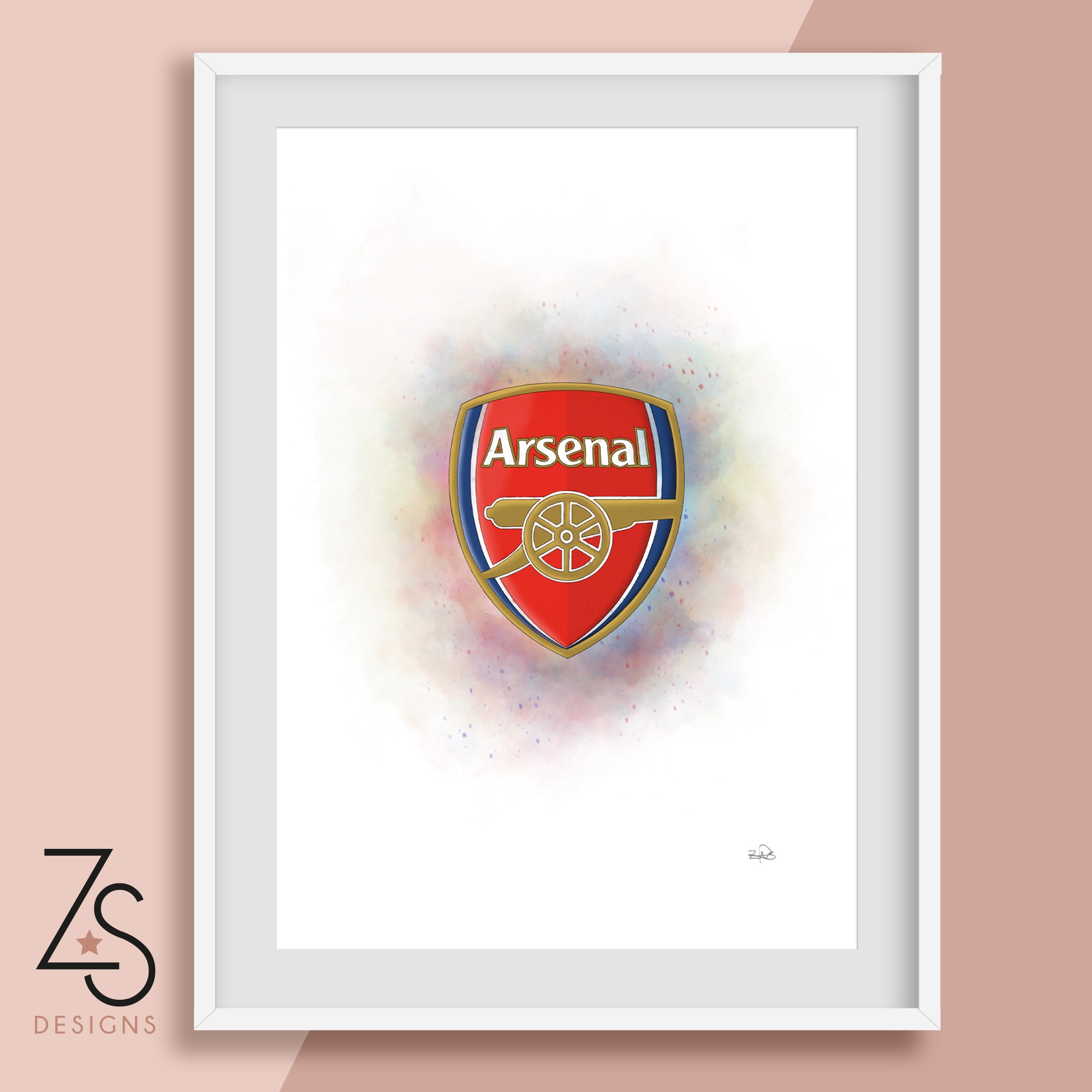The image showcases a product by ZS Designs, set against a two-toned pink diagonal background, with light pink on the top left and darker pink on the bottom right. Positioned in the bottom left corner, the ZS Designs logo features a diagonally-styled "Z" and "S" forming a triangle, with a mauve star at the intersection and the word "DESIGNS" in all caps below. Dominating the center of the image is a virtual or possibly real framed photograph of a sports team logo, with a silver, off-white, and light bluish frame. The focal point inside the frame is the emblem of Arsenal FC, featuring a bold white "ARSENAL" in gold-rimmed font on a red shield. The shield, divided into two red tones, carries a yellow cannon with a six-rimmed wheel. The logo is overlaid on a pale watercolor splotch of various pastel hues, with the entire composition against a white background. A small cursive signature in the bottom right corner of the photograph adds a touch of authenticity, rounding off this detailed graphic design mock-up.